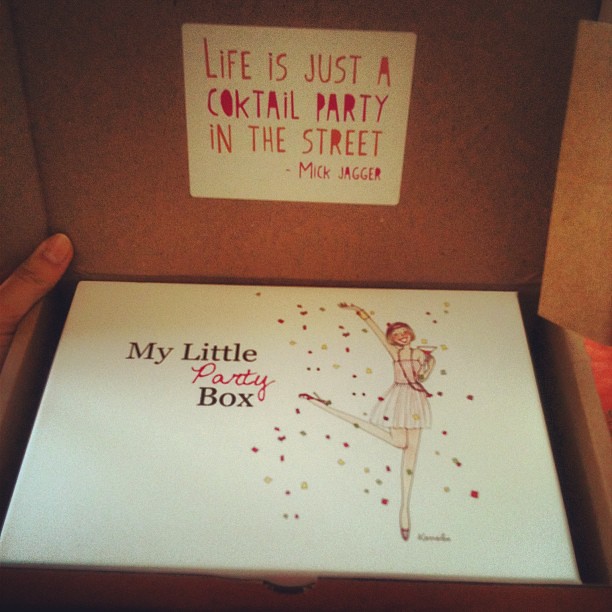The image captures a person opening a cardboard box, using their thumb to hold the cover open, revealing another smaller white box inside. The outer cardboard box features a sticker on the inside of the cover that reads, "Life is just a cocktail party in the street" attributed to Mick Jagger, written in a vibrant red font over a white background. The inner white box has a festive illustration of a woman in a celebratory pose, standing on one leg with one arm raised, holding a drink that appears to be a margarita. She is adorned in a short pink dress, high heels, a little hat, and a long red necklace, with confetti in red, gold, and silver sparkling around her. The box is labeled "My Little Party Box" where "party" is written in a playful red cursive font, contrasting with the more traditional black Times New Roman font used for the rest of the text. The overall scene suggests a fun and festively themed package, likely promising something delightful inside.